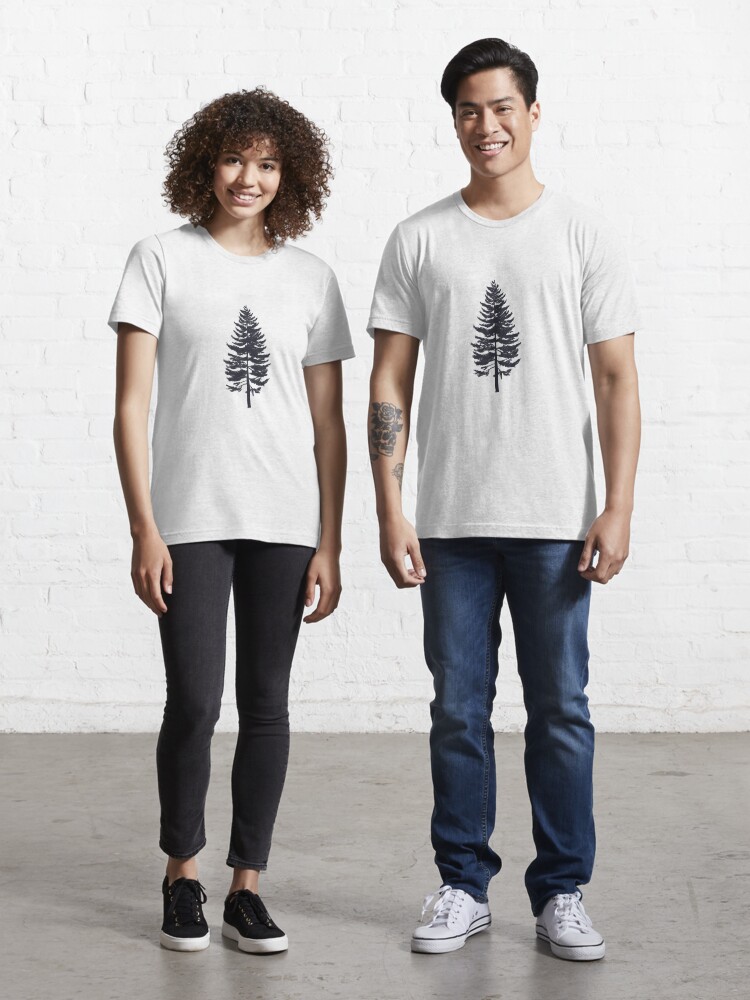This is a detailed portrait photograph of two people, a woman and a man, modeling matching T-shirts in front of a white brick wall. The man stands on the right side and the woman on the left. The woman has very curly, dark brown hair that reaches just above her shoulders and she is smiling at the camera. She is wearing black yoga pants and black Converse sneakers with white trim. The man has neatly combed black hair and he is also smiling. He is wearing blue jeans that are slightly too long, covering part of his white sneakers with blue trim. Both are dressed in identical cream-colored T-shirts featuring a black-shaded pine tree design in the center. The man has a visible tattoo of a skull with an intricate headpiece on his right forearm. They are standing on a grey cement floor, and the overall setting suggests an indoor location with a minimalist style.